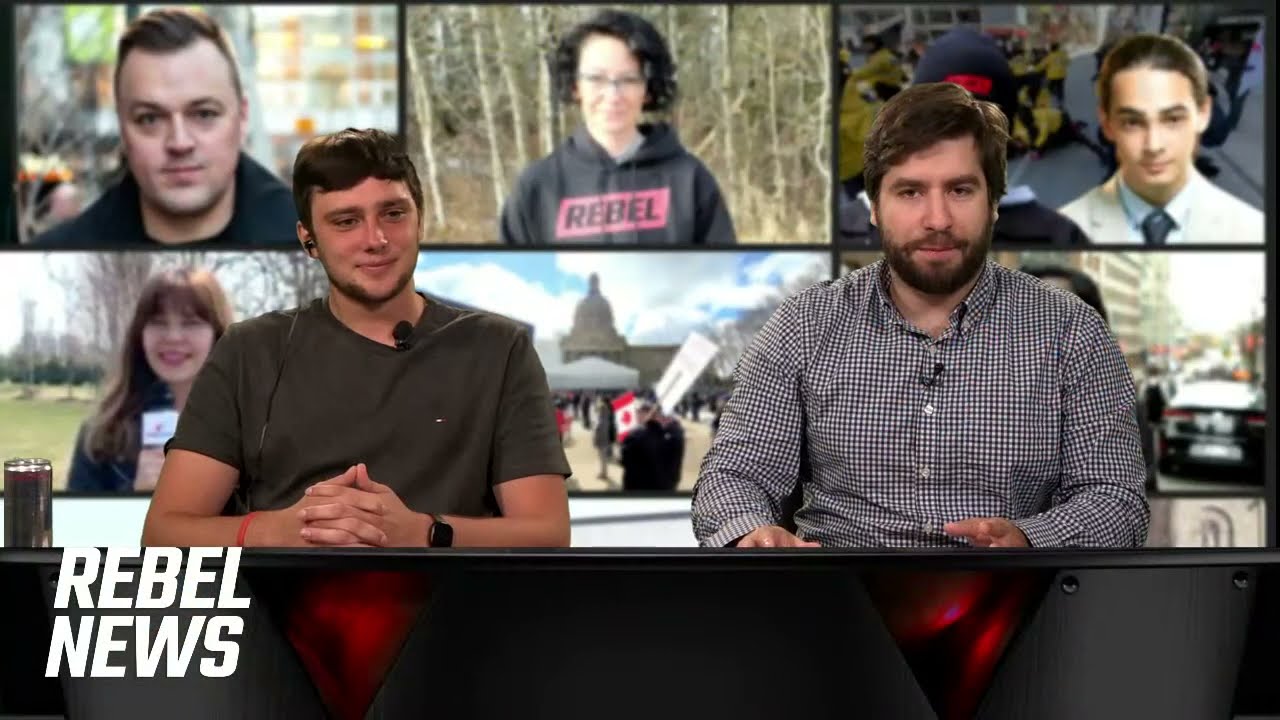The promotional image, attributed to Rebel News and identifiable by the bold white text in the lower left corner, showcases two men casually sitting at a table, both equipped with microphones and earpieces. The man on the left, sporting a short-sleeved olive shirt, short brown hair, tanned skin, a red bracelet, and a watch, appears to be slightly smirking. Beside him, another man with short brown hair and facial hair dons a long-sleeved black and white checkered button-down shirt. In the background, there is a screen displaying six distinct images: a man in a black jacket looking towards the camera outdoors, a woman in glasses wearing a "Rebel" hoodie, another man in a lab coat, a woman holding a microphone, an image of a large building, and a picture of a car. The overall color scheme of the image includes shades of black, white, gray, brown, olive, red, and silver. The scene paints a vivid picture of an informal news reporting setup, with various visual elements highlighting the diverse team behind Rebel News.